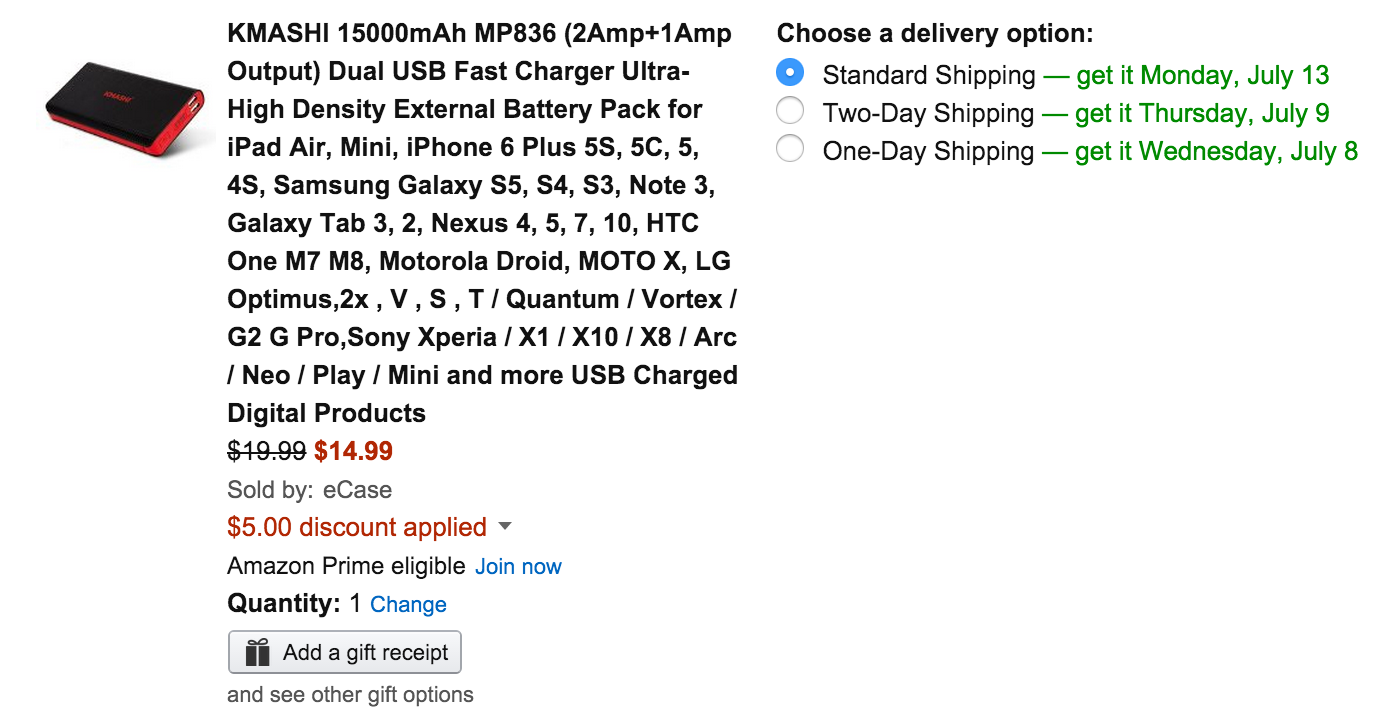Listing for a Kmashi 15,000 mAh MP836 Dual USB Fast Charger

This ultra-high-density external battery pack, suitable for a wide range of devices including iPad Air, iPad Mini, iPhone 6 Plus, and iPhone 5s, boasts a powerful 15,000 mAh capacity with 2A and 1A output ports for efficient charging. Previously priced at $19.99, it is now available for $14.99 with a $5 discount applied. Sold by e-case, this product is eligible for Amazon Prime, inviting you to join for additional benefits. The listing displays a 'Quantity: 1' option with the ability to change the amount or add a gift receipt. Three shipping options are offered: standard shipping with an estimated arrival by Monday, July 13th, two-day shipping, or one-day shipping. The shipping dates are prominently highlighted in green for easy reference.